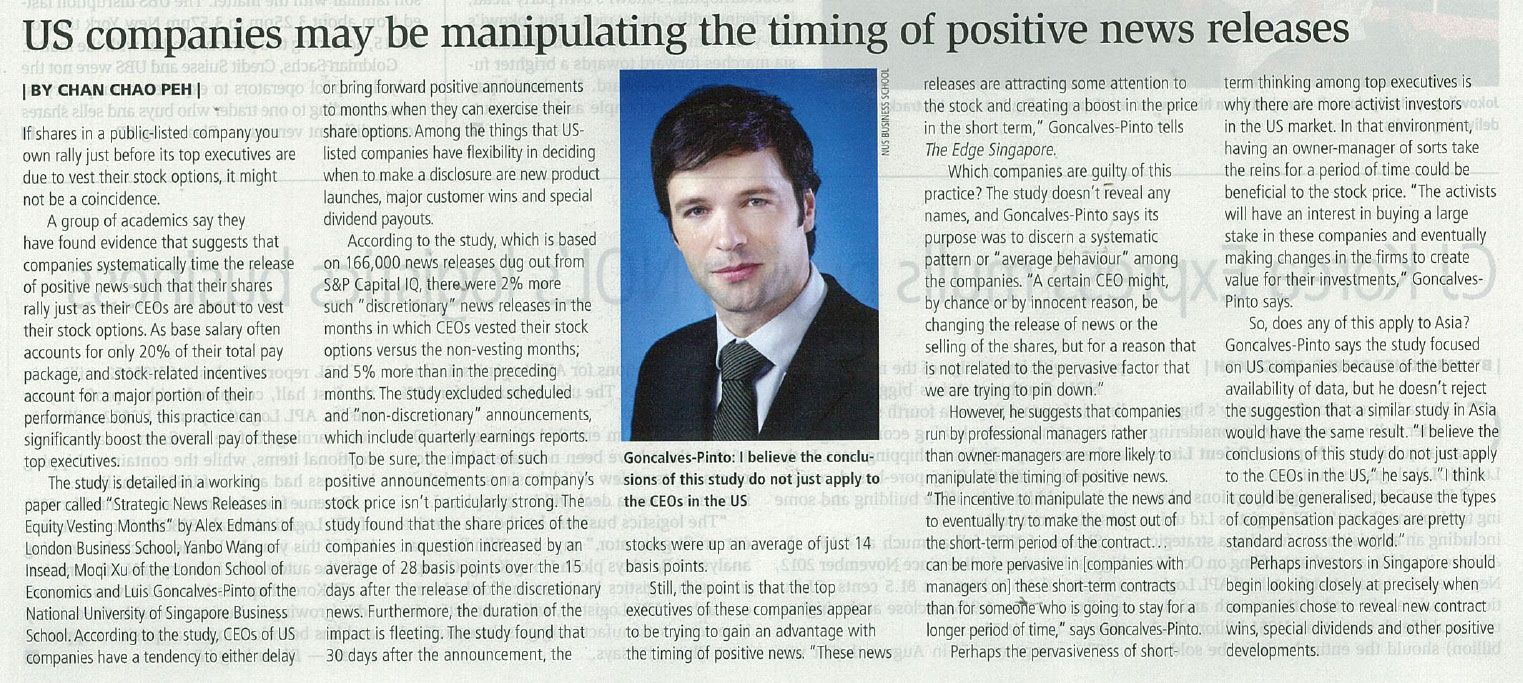**Title: U.S. Companies May Be Manipulating the Timing of Positive News Releases**

Authored by reporter Chen Chaofan, this newspaper article spans five columns, delving into the strategic timing of corporate news releases. Dominating the middle column's top half is a photograph of a man adorned in a suit and tie, identified as Goncalves Pinto. Accompanying the image is his quote: "I believe the conclusions of the study do not just apply to the CEOs in the U.S."

The article opens with a compelling assertion: "If shares of a publicly listed company you own rally just before its top executives are due to vest in their stock options, it may not be a coincidence." A group of academics claims to have unearthed evidence indicating that companies systematically time the release of positive news, aligning it with the vesting of CEOs' stock options. This strategic release of news can significantly inflate the overall compensation package of top executives, given that their base salary typically constitutes only about 20% of their total remuneration, with stock-related incentives forming a substantial portion of their performance bonuses.

The body of the article meticulously outlines the various mechanisms and schools involved in studying this phenomenon, presenting a detailed investigation into the practices of news release timing. Concluding with implications for investors, the final paragraph advises that "perhaps investors in Singapore should begin looking closely at precisely when companies choose to reveal new contract wins, special dividends, and other positive developments."